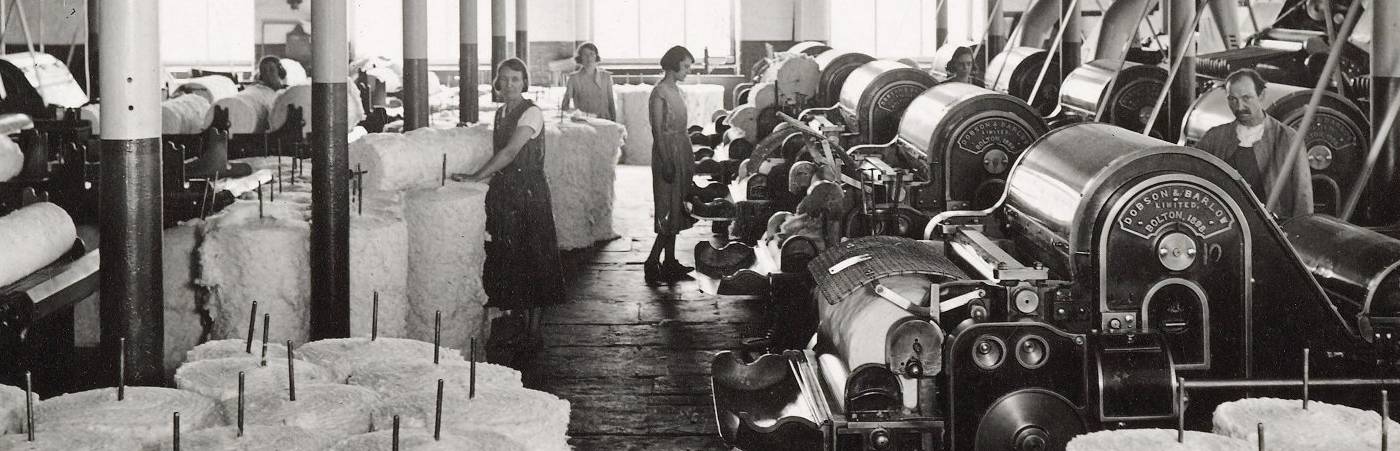In this black-and-white panoramic photograph, taken likely between the 1920s and 1940s, we are inside a bustling textile factory filled predominantly with women workers. The women, all wearing long dresses with their hair styled to chin-length, are diligently operating and monitoring large, intricate machines. These impressive machines, lined up in two parallel rows, have a distinctive shape with a rectangular body and a pronounced curved top, resembling the silhouette of a Volkswagen. They are processing hefty white bolts of material, possibly bolts of fabric or yarn, which some of the women are seen handling with care, loading them onto the machines to ensure continuous operation. One man, an older worker with a receding hairline and a mustache, stands discreetly in the background between the rows of machines, overseeing the factory floor. The detailed image captures the essence of early industrial textile manufacturing, highlighting the vital role of women in this labor-intensive environment.